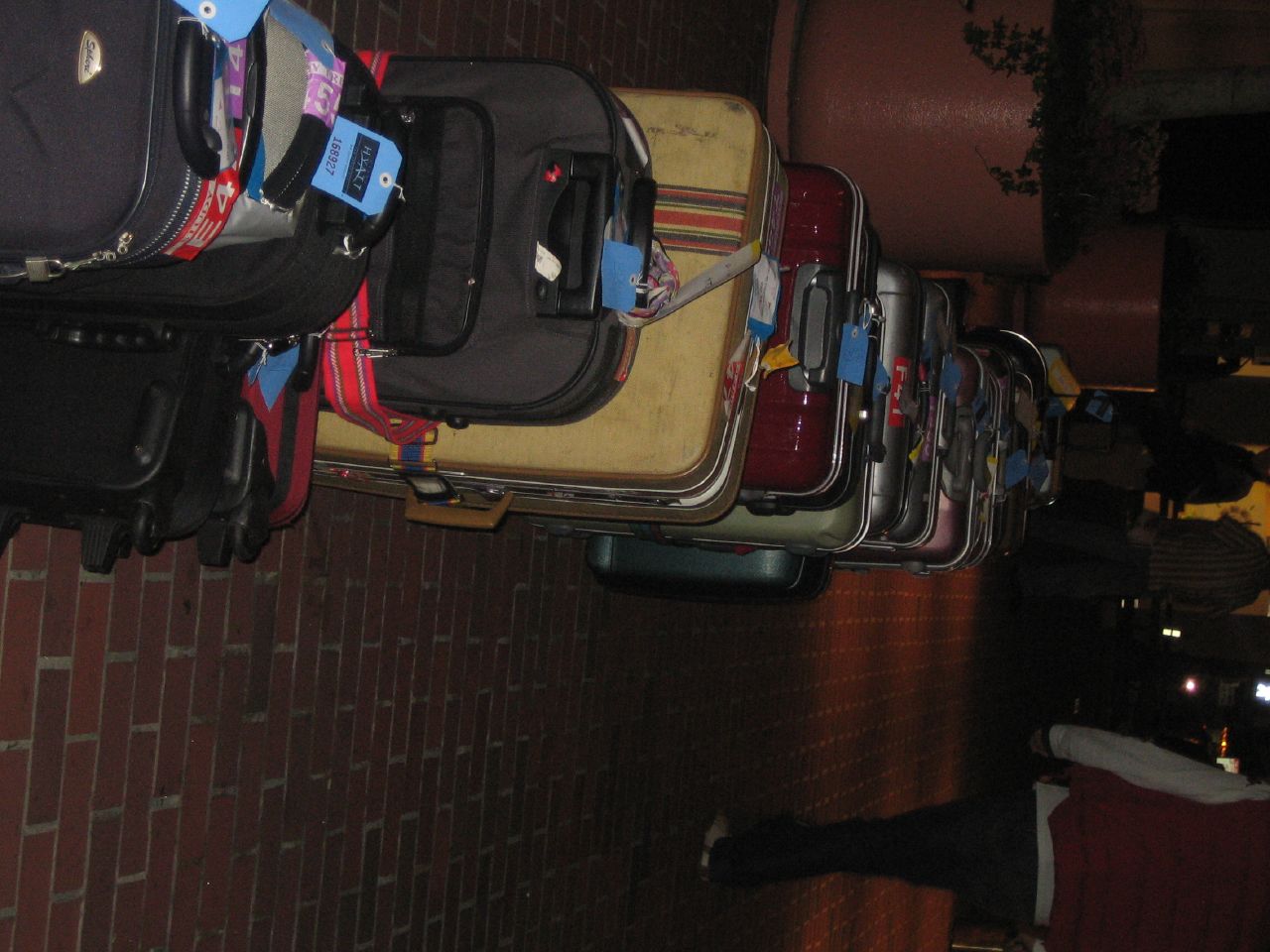In this color photograph, which is predominantly dark with a palette of deep browns and intermingled hues, we see a long line of various suitcases extending from the bottom left corner to almost the top of the image. The suitcases, resembling a row of leaning dominoes, vary in size and style, ranging from modern rollaway luggage to vintage 1960s cases. Notable colors include black, yellow, red, green, beige, and some with stripes. A blue tag is visible on at least one of the bags. These suitcases are situated on a brick floor comprising bricks of dark red to light red, with grayish mortar between them.

To the left of the luggage is a large terracotta planter with indistinguishable foliage, dark due to the nighttime setting. Another similar planter is seen further along the left-hand side. The upper part of the image is dark, with lines of light visible towards the top of the bags. 

In the upper right-hand corner, a person is walking away, dressed in black trousers, a reddish vest, a grayish or whitish top, and possibly black and white shoes. Their head is cut off from the frame. To the right of this person are some indistinct streetlights, contributing to the dim lighting of the scene. Further in the background, several people are standing near another large planter, with a yellowish backdrop and white lights, adding depth to the composition.